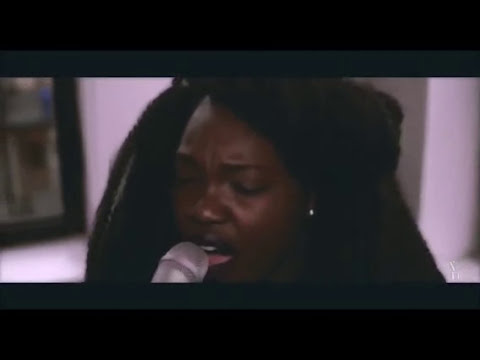In this image, a black woman with long, thick, black hair is passionately singing into a silver-colored microphone. Her eyes are closed, and her mouth is open, revealing her white teeth and pink bottom lip, suggesting she is deeply engrossed in her performance. The woman is centered in the frame, with the microphone positioned in front of her mouth. She appears to be indoors, as the blurred background reveals a white wall with a painting and possibly a black-framed window to the left. There is also a white cylinder column, which looks like it's made of cement, and a glimpse of a white floor, hinting at an indoor setting that could resemble a store or a house. The image has black and blue strips at the top and bottom, reminiscent of a movie theater screen or a video aspect ratio, adding a cinematic quality to the scene. The woman's left ear features an earring, adding a touch of personal style to her expressive performance.